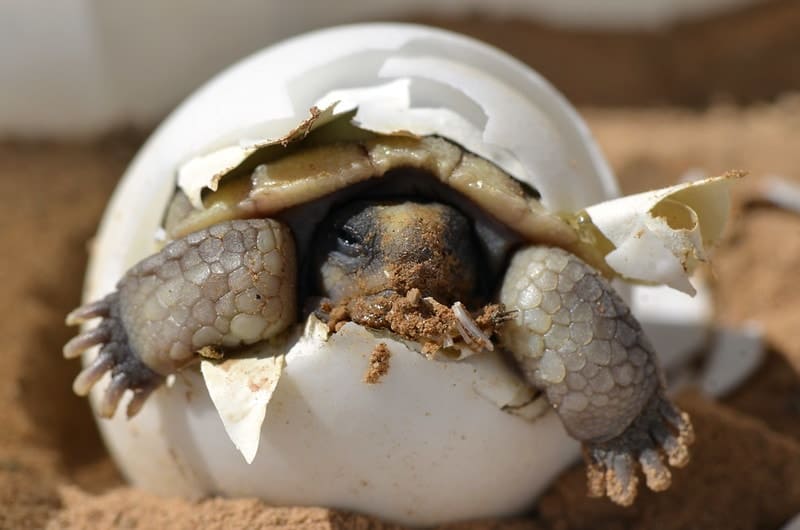A professionally taken, horizontally rectangular, full-color photograph captures the remarkable moment of a baby sea turtle emerging from its shell, set against a blurred sandy background. The natural daylight illuminates the scene, highlighting the baby turtle’s textured, light gray scales and its partially open eyes as it digs its way out. The turtle's front legs, adorned with subtle round patterns, protrude from the shell, with some dirt visible on them, especially on the left one. The shell itself, predominantly intact, has a noticeable break on one side where the turtle is making its exit, with fragments scattered on the sandy ground to the right. Other white splotches at the top of the image likely indicate additional turtle eggs. The backdrop of rough, freshly dug sand emphasizes the turtle's emergence in this intimate nature study.